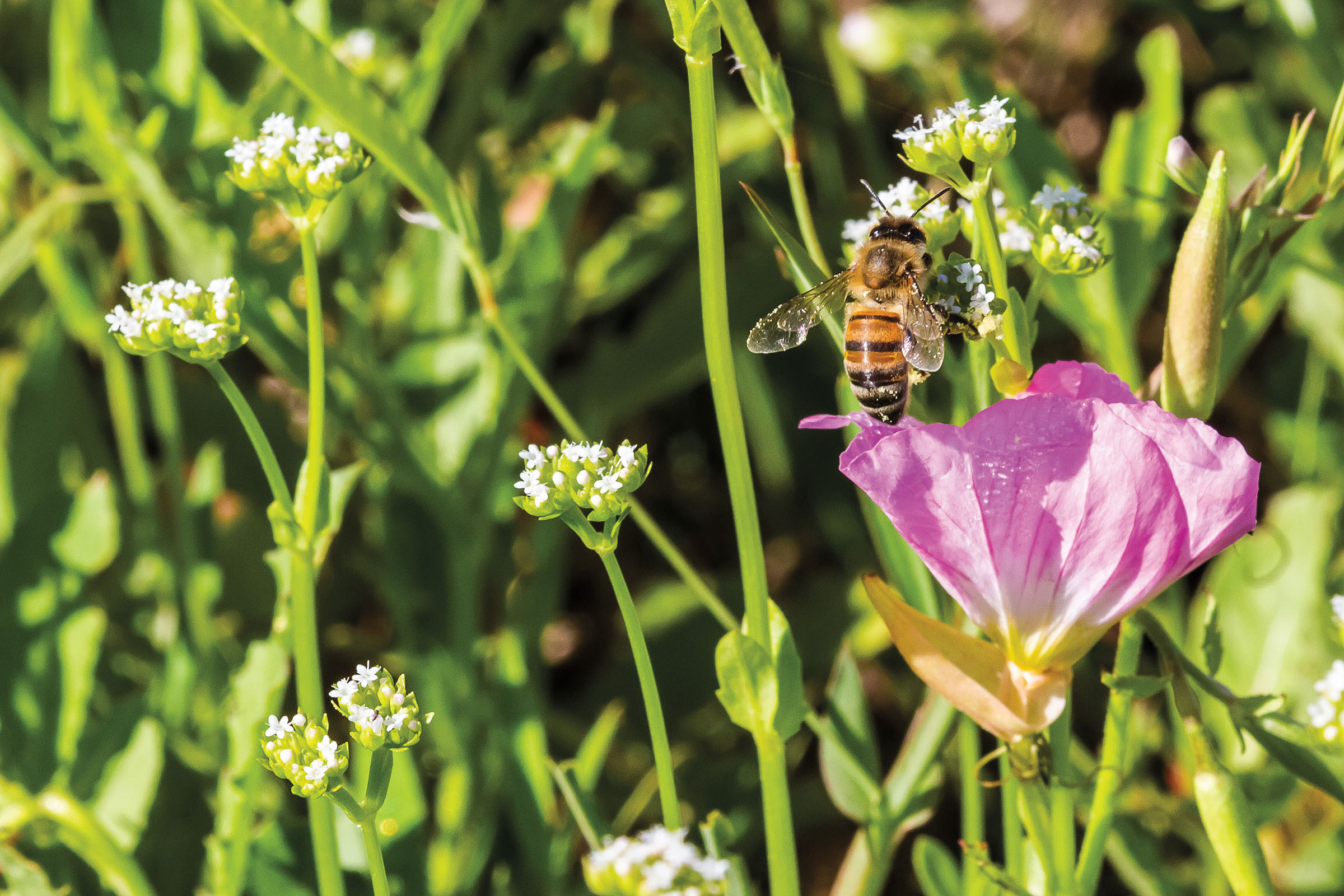In this vivid photograph of nature, we see an intricate scene dominated by green stems topped with tiny white flowers in full bloom. The focal point to the right of the image is a large pink flower, which, though no longer in its prime, still adds a touch of color despite starting to fold in on itself and showing hints of browning. The photo captures a busy bee, characterized by its golden and black striped body and fuzzy head, diligently gathering pollen from the white blooms. The bee’s delicate translucent wings and tiny antennae are also noticeable, adding to the rich detail of the image. The interplay between the green stems, the white flowers, and the pink flower—alongside the industrious bee—paints a beautiful and complex picture of a moment in nature.